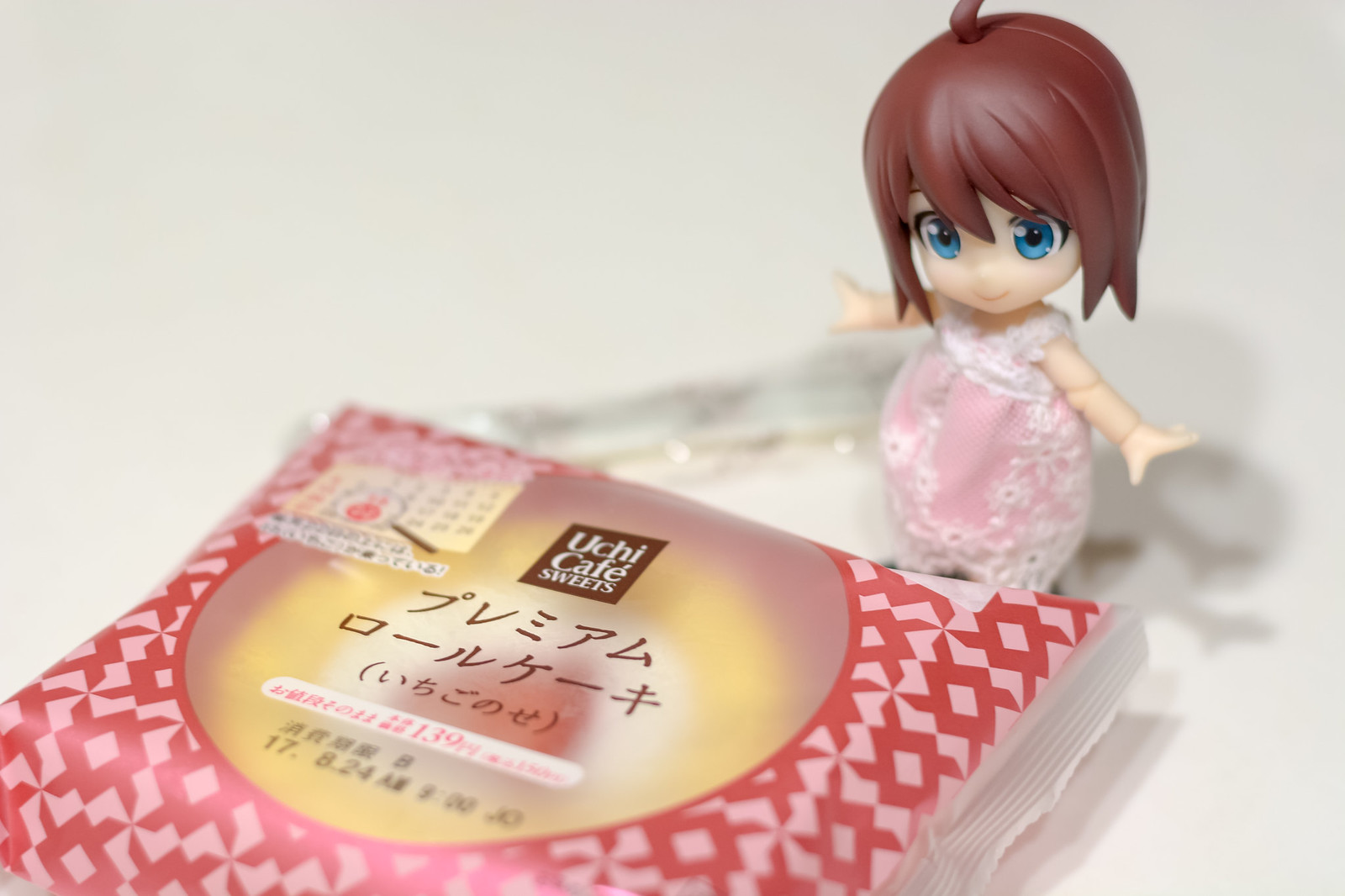The image showcases a small figurine of a girl and a packaged pastry on a white background. The figurine, resembling an anime-inspired doll, stands to the left of the pastry. The doll is dressed in a pink and white dress with her arms outstretched, displaying her big blue eyes, tiny nose and mouth, and dark brown hair. The pastry is enclosed in a pink and red plastic bag, tilted at an angle, with a clear middle section revealing a beige, white, and red dessert inside, possibly a cake or Danish. The packaging features a brown box at the top with the inscription "UCHI CAFE SWEETS" in white text, along with some additional Japanese writing. The detailed packaging design includes white pinwheels and a yellow circle. Overall, the scene is meticulously arranged to highlight both the figurine and the pastry, creating a charming and whimsical display.